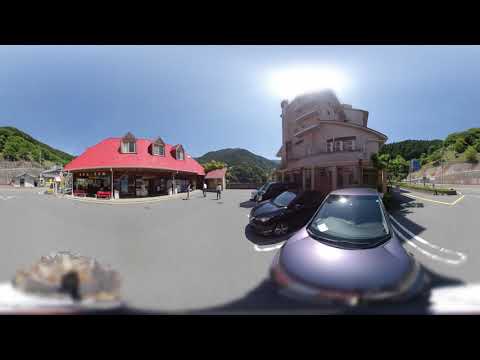The image depicts a distorted, close-up view from a wide-angle or fisheye lens, possibly from a dash cam. Dominating the foreground is a bluish-purple car with a rounded, distorted shape due to the lens effect. White parking lines are clearly visible on the grey ground. Behind this car, there is a black vehicle.

The cars are parked in front of a brown or greyish-white, irregularly constructed building that stands about three stories tall, occupying the right side of the image. Its design appears disproportionate and lacks defining signs.

On the left side of the image, there's a building with a red roof and three dormer windows, suggesting it might be a shop, market, or general store. Near its entrance, three people are seen standing. Behind this building, there's a small shed.

The background is adorned with three small, tree-covered hills that span from the left to the right of the image, contributing to the scene's natural setting under a clear, blue, and sunny sky.